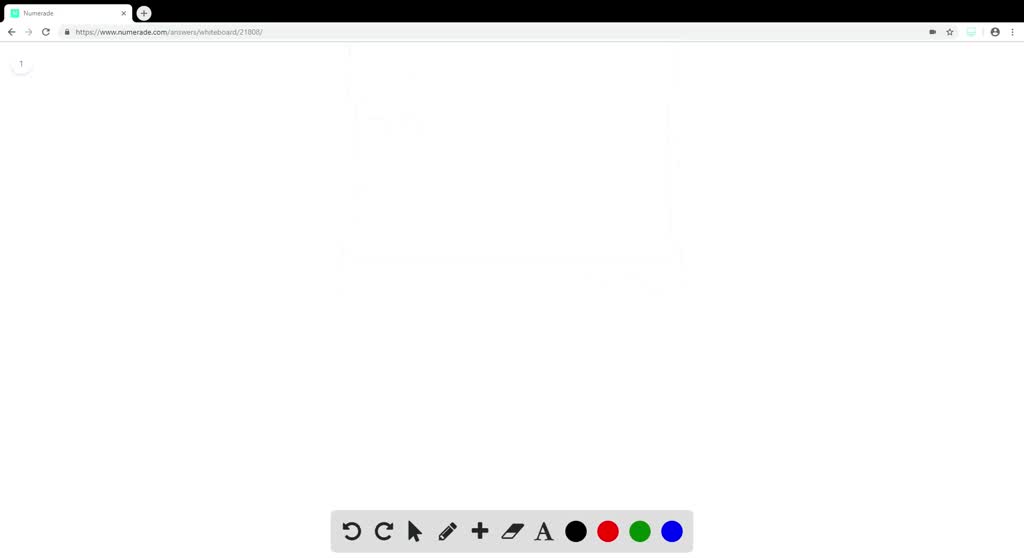In this screenshot, we observe a predominantly white webpage displayed from the website https://www.numeraid.com. Positioned in the upper left corner of the image, the browser window highlights the URL in the address bar, a small green box to its left, and a left-pointing arrow icon that is highlighted, indicating a previous page or navigation option. Immediately beneath the address bar, the page is enumerated with the number "1" situated on the left side. 

At the bottom of the image, a gray toolbar provides various functionalities. From left to right, the toolbar features an assortment of icons: a left-pointing arrow, a right-pointing arrow, an arrow pointing diagonally to the upper left, a pencil icon, a plus sign, a letter “A.” Further to the right are four circular color options arranged sequentially as black, red, green, and blue.